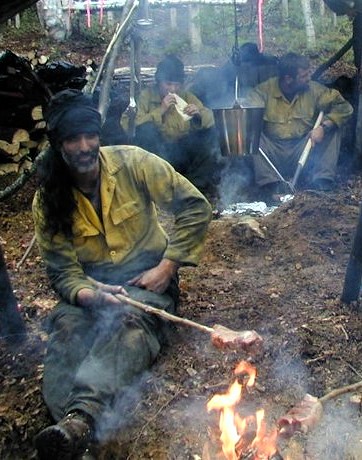The photograph captures a group of men cooking outdoors in a dirt-covered area, surrounded by small rocks and twigs, possibly in a forested setting. In the foreground, a man is seated on a pile of dirt, wearing dark, almost black pants and a dirty yellow long-sleeved collared shirt. He has a black turban wrapped around his head, with long hair cascading down to his chest, and he sports a full beard. Holding a stick with a piece of meat over an open fire, he appears deeply engaged in cooking. To his right, another stick with meat hovers over the fire, although the person holding it is out of frame. 

In the background, at least two other men are also sitting on the ground, wearing similar yellow shirts and dark pants. One of them is stoking the fire beneath a pail, causing smoke or steam to rise, while the other is biting into a piece of whitish bread. Scattered around them are a few firewood pieces, adding to the rustic, makeshift cooking scene. The backdrop reveals some trees and foliage, suggesting a forested area. The overall atmosphere hints at a group living in modest conditions, gathered for a communal cooking experience.